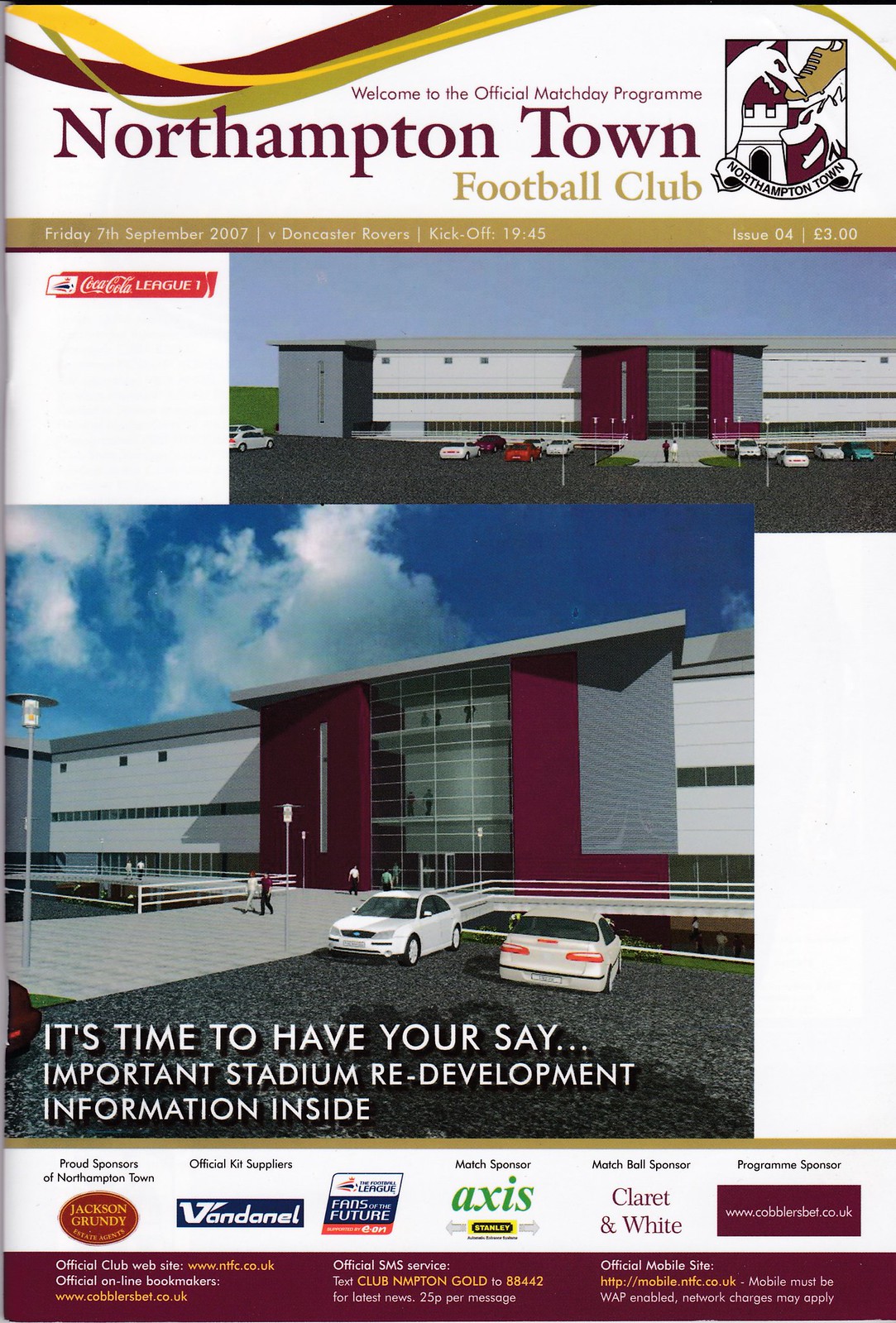The image is the cover of a match day program for Northampton Town Football Club, delineated by swirling yellow, burgundy, and green patterns at the top. Prominently featured at the top center is the text, "Welcome to the Official Match Day Program, Northampton Town Football Club," with a team crest to the right displaying a lion, a wolf, a soccer shoe, and a castle. Below the crest, a tan bar provides the details: "Friday, 7th September 2007, V. Doncaster Rovers, Kick-Off 19:45, Issue 04, £3."

The main section of the cover features two images of a large white building with a striking red entrance, likely representing the club's stadium renderings. The first shows the building from one angle, while the second image presents another perspective with two white cars parked in front and several people walking around. A Coca-Cola League emblem is noted in the top left of this section.

At the bottom, text invites readers to engage: "It's time to have your say. Important stadium redevelopment information inside." Additionally, a list of sponsors, including sports businesses and travel agents, is displayed.